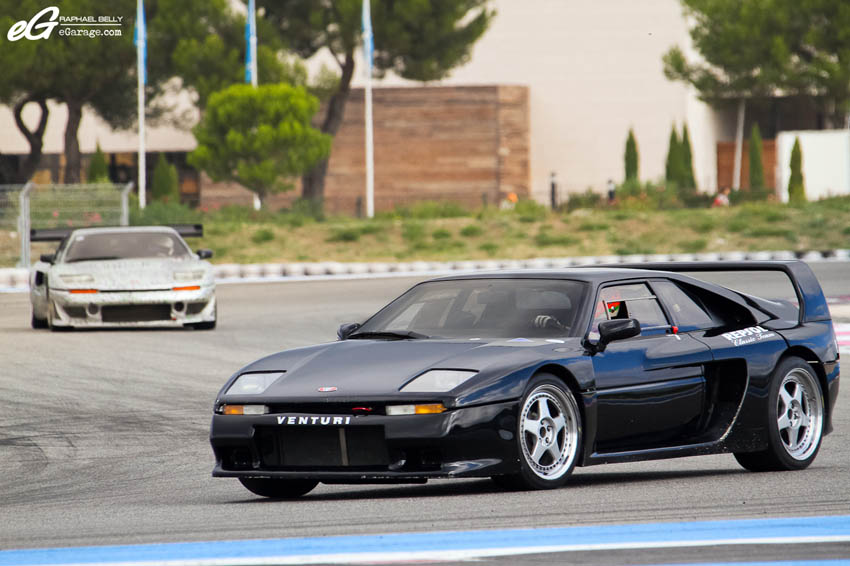The image shows two race cars on a grey racetrack, set against an outdoor background featuring some trees and flagpoles with blue flags. The car closer to the camera on the right side is a black race car with the word "Venturi" boldly displayed in white on its front bumper. This car, which has a large raised spoiler on its back and silver alloy rims, resembles a Mazda 300X. A man inside it is visible, with his hand on the steering wheel. To the left, there's a grey race car distinguishable by its orange accents below the headlights and a black spoiler. Both cars seem like older models, potentially from the 80s or 90s. The racetrack features blue and white stripes on its surface. In the blurred background, there's a large white and brown building partially hidden by trees, as well as other smaller trees. A gate or fence is visible on the left along a curve of the road, adding to the scene’s depth and context.